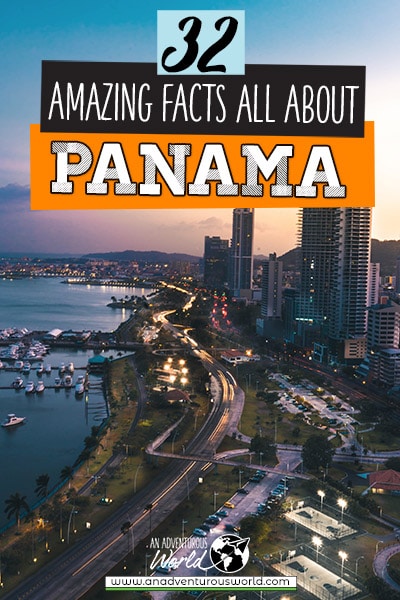The poster features a vibrant city skyline at dusk, with a waterway and a busy thruway lined with vehicles that appear as streaks due to motion blur. The skyline includes a mix of hotels and office buildings, capturing the bustling essence of the city. On the waterway, several small sailboats are visible, adding a serene touch to the scene. The foreground also reveals basketball and tennis courts, indicating a lively recreational area.

At the top of the poster, within a square box, the number "32" is prominently displayed. Beneath it, another black square box contains the text "Amazing Facts All About." Following this, in bold orange letters, is the word "Panama." Below, the slogan "An Adventurous World" is inscribed, accompanied by an image of a globe. The website www.anadventurousworld.com is printed at the bottom, guiding viewers to learn more about the intriguing facts presented.

The overall composition, including the dynamic interplay of the vehicles on the thruway, the peaceful boats on the waterway, and the glowing skyline, perfectly encapsulates the allure of Panama at sunset.